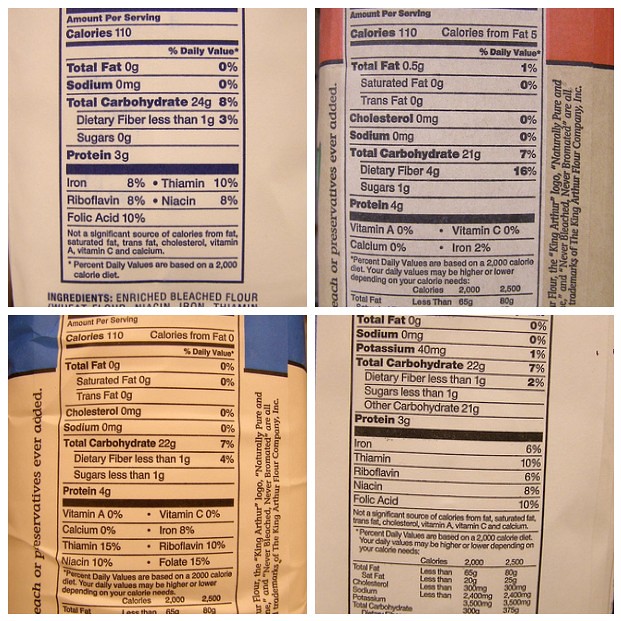This image is divided into four quarters, each showcasing the nutrition labels from various types of flour. 

In the top left quarter, the flour contains 110 calories and 24 grams of carbohydrates per serving. It also provides 10% of the daily value (DV) for folic acid, 8% for riboflavin, niacin, and iron, and 10% for thiamine. 

The bottom left quarter features a flour with 110 calories and 22 grams of carbohydrates per serving. Notably, it has no vitamin A, calcium, or vitamin C. However, it offers 8% DV for iron, 15% for thiamine, 10% for niacin and riboflavin, and 15% for folate.

In the top right quarter, the flour also has 110 calories but 21 grams of carbohydrates per serving. It lacks vitamin A, vitamin C, and calcium, while providing 2% DV for iron.

The lower right quarter shows a slightly obscured label where the calorie count isn’t visible. This flour includes 22 grams of carbohydrates and 40 milligrams of potassium per serving. It offers 6% DV for iron and riboflavin, 10% for thiamine and folic acid, and 8% for niacin.